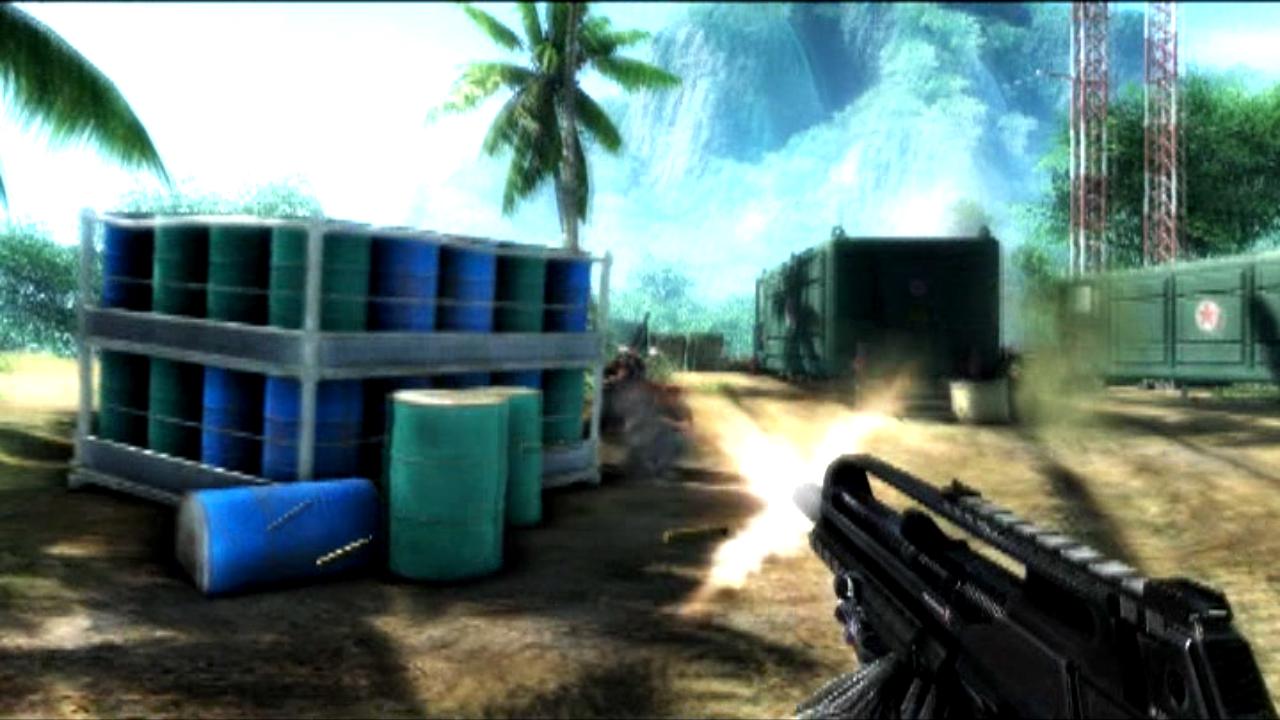The image depicts an intense on-screen gameplay scene. In the foreground, a black machine gun is being fired, with a bright muzzle flash illuminating the area. Directly ahead, a stack of barrels, enclosed in a gray cage, come into view. The barrels are painted green and blue, meticulously arranged in two tiers of 20 barrels each — the bottom row comprising 20 barrels, and an identical set stacked on top. Outside the cage, two additional barrels are visible. In the distance, the sky is filled with dense smoke, partially obscuring a rugged, mountainous landscape reminiscent of an Ice Age setting.